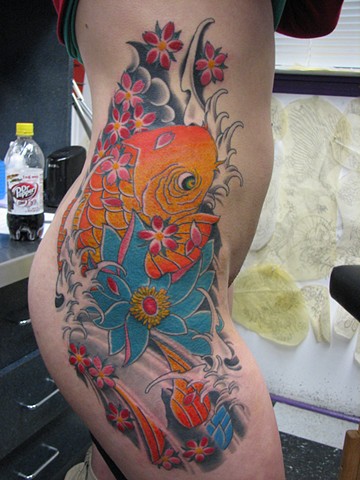The image captures the right side of a relatively pale, white man showcasing an elaborate and colorful tattoo that spans from the upper torso, across the side of his butt, down to just above the knee. The intricate tattoo features an orange koi fish adorned with detailed scales, accompanied by large blue and green flowers, several small red and orange flowers, and an artistic wave pattern in the background reminiscent of Japanese style. The man is standing in front of a clear window with a black cabinet behind him, featuring black drawers and a Dr. Pepper bottle placed on top. The setting appears to be indoors, possibly in a bathroom or a tattoo parlor, as there are cabinets and a window visible in the background. No genitalia is shown, and the overall image focuses on the vibrant tattoo as the central element.